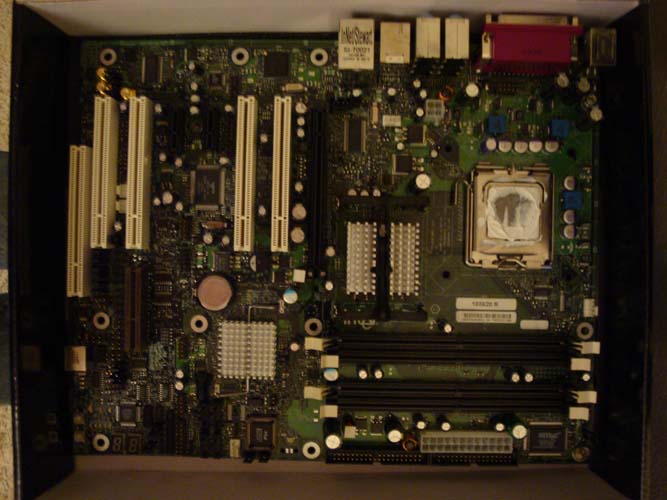This detailed photograph captures an overhead view of a computer motherboard, presumably positioned inside an open cardboard box. The green printed circuit board (PCB) stretches to fill the entire frame. On the upper left-hand corner, five thin yet tall expansion slots are visibly aligned. Moving to the lower right, four RAM slots and the main power connector are prominently situated. Central to the image, two distinct bridges, each adorned with a silver heatsink, take a prominent position. Adjacent to these, on the center-right, is the processor slot. The motherboard's inputs and outputs are found in the upper right-hand corner. Additionally, a small battery and various connectors are dispersed throughout, making the motherboard resemble a miniature, intricate electronic city. The motherboard appears slightly wider than it is tall from this perspective.